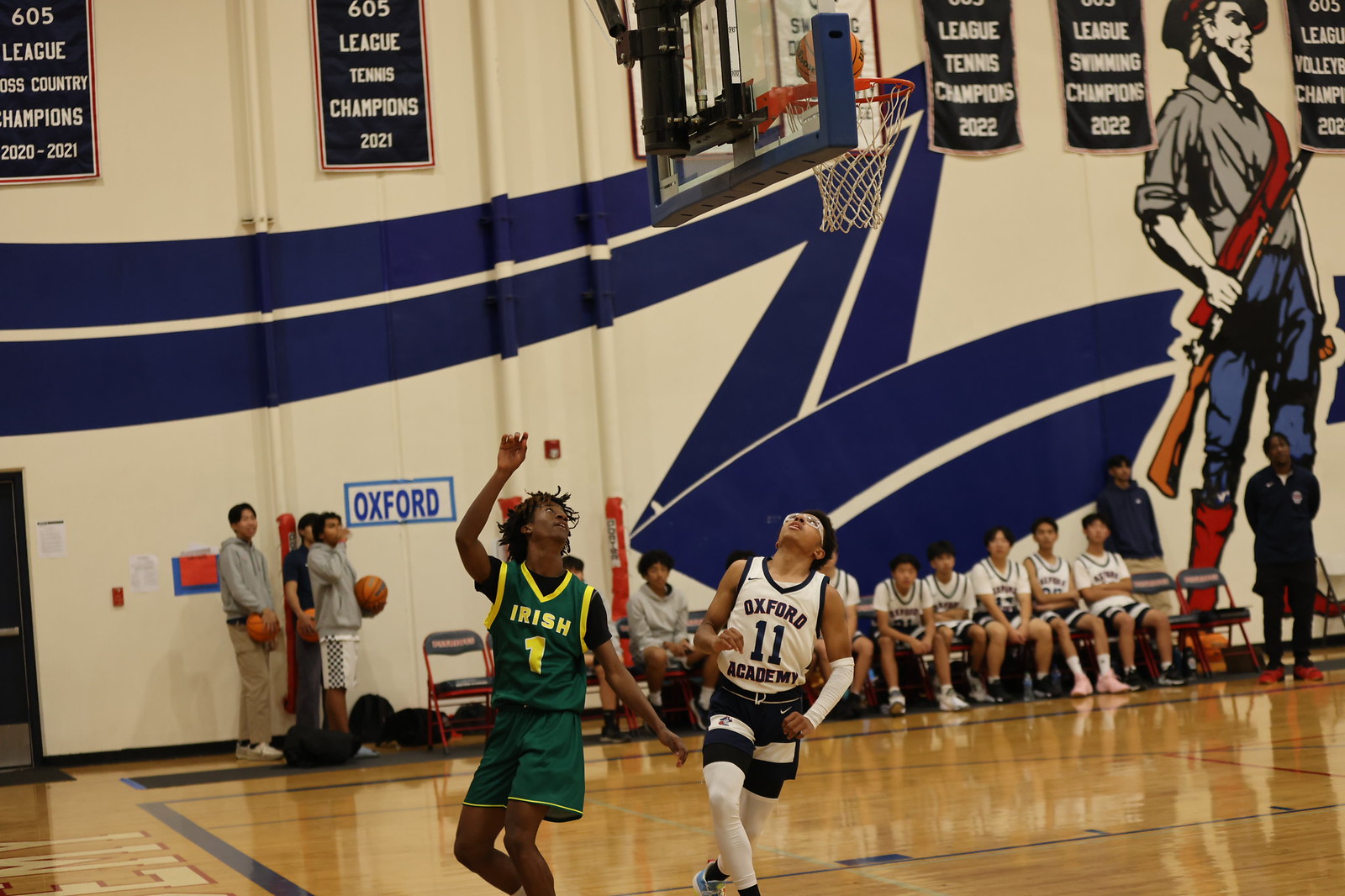The image depicts a high school basketball game inside a gymnasium. Central to the scene are two players beneath the basketball hoop with a ball poised above the rim. The player shooting is wearing a green jersey with yellow trim that says "Irish," and he's identified as number one. He is a Black athlete with dreadlocks. To his right is a player from the opposing team, Oxford Academy, wearing a white jersey with blue stripes, number 11, and protective goggles. This player appears to be either Black or Asian. 

Behind the players on the court, a bench is filled with athletes from Oxford Academy, all donning similar white uniforms with blue accents. Spectators and additional players are visible, with some standing and holding basketballs. The gym's walls display numerous banners celebrating league championships in various sports like cross country, tennis, and swimming. A noticeable feature is a large mural of a warrior, signifying Oxford Academy's mascot, along with blue lines. A blue box on the left side of the wall, bearing the name "Oxford," confirms they are the home team.